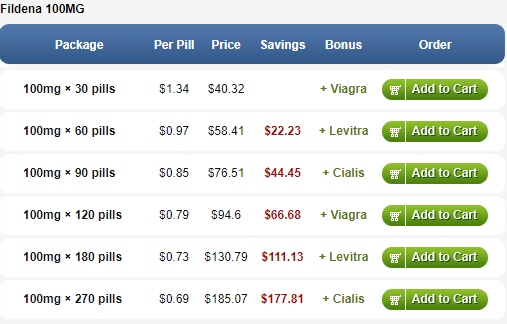The image depicts a detailed screenshot of an e-commerce website showcasing a product menu with pricing information for Faldina 100 milligram pills. The menu is presented on a white background and features a blue border that divides the content into six columns: "Package," "Per Pill Price," "Price," "Savings," "Bonus," and "Order."

In the top left corner, the title "Faldina 100 milligrams" is displayed. Below the title, each row within the columns provides detailed information on different purchasing options for the pills. The first row lists 100 milligrams x 30 pills with a per pill price of $1.34, a total price of $40.32, no savings, and a bonus of free Viagra pills. Each subsequent row follows a similar format with varying quantities:

- 100 milligrams x 60 pills
- 100 milligrams x 90 pills
- 100 milligrams x 120 pills
- 100 milligrams x 180 pills
- 100 milligrams x 270 pills

The per pill price decreases as the quantity increases, with the lowest per pill price being $0.69. The total price range for these packages varies from $40.32 to $185.07. Each option includes different bonus pills, such as Viagra, Levitra, and Cialis. 

To the right of each bonus offering is a green "Add to Cart" button for easy purchasing. The layout effectively organizes the information, allowing users to compare different buying options at a glance.